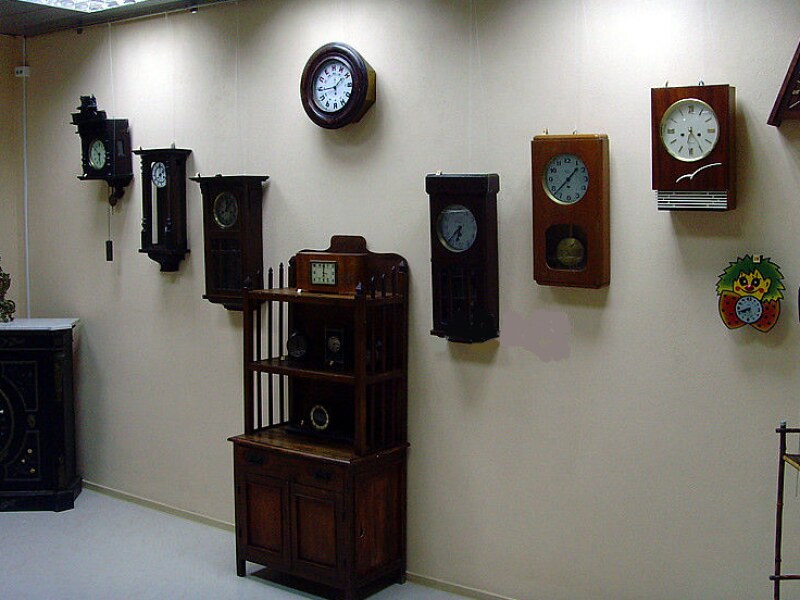The image depicts an interior space, possibly a home or museum, featuring a horizontal rectangle-shaped wall adorned with various analog clocks. The background wall is a light beige or cream color, complemented by a light gray floor and a dark gray ceiling with overhead lights that illuminate the scene. The clocks, numbering at least eight, are free of digital elements, showcasing traditional white faces with black numerals or Roman numerals, and some just have lines to denote time.

Dominating the composition, the clocks are crafted from various wood types including dark oak and lighter woods. One distinct clock has a whimsical clown face with green hair, yellow skin, blue eyes, and is adorned with a red and black polka-dot bow beneath its face, where the clock hands are positioned. 

At the top center of the arrangement is a round clock, and directly below it is a cabinet featuring an integrated clock. This cabinet sits slightly elevated from the ground. The clocks extend outward from the center in a formation resembling a broad "V", with their arrangement curving from the top left down to the bottom center and back up to the top right. 

In the far left corner, there is a small, intricately designed mini curio cabinet made of dark wood, possibly black, with a white marble top. Additionally, towards the right side of the image, another wooden cabinet with shelving and a clock integrated into its structure can be seen. This setup gives the impression of a curated, almost gallery-like display of timepieces.